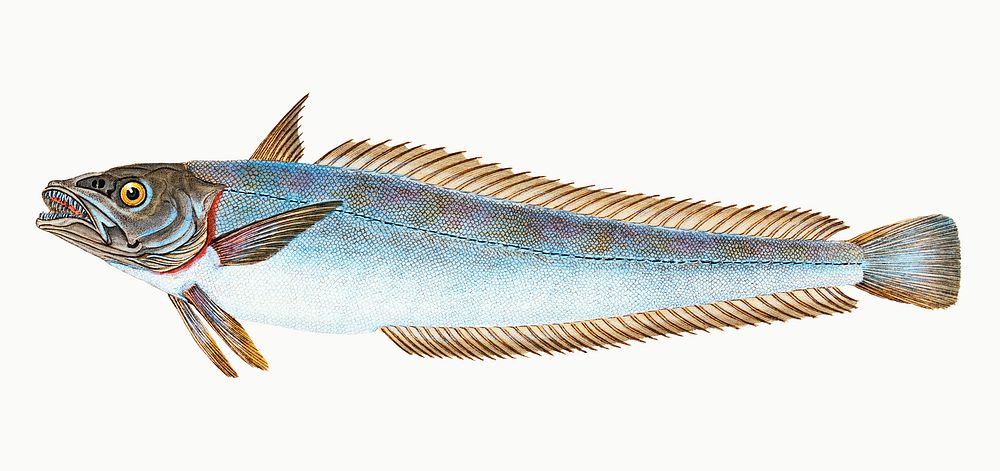This detailed professional art print or colored pencil drawing features a large, elongated fish set against an off-white or very light gray background, emphasizing its intricate design. The fish is adorned with a blend of blue hues and brown speckles, particularly on its upper body, transitioning to lighter blue and white towards its belly. Noteworthy are its brown fins, including two prominent ones near its front, a series of smaller fins along its back and belly, and a shorter tail fin with blue and brown coloration. The fish’s head is darker gray with striking yellow eyes, accented by sharp, blue-tinged teeth reminiscent of a gar. Red highlights can be observed around the gill area, adding depth. A distinct line runs from the gills along its length to the tail, coupled with spines on its back that add to the fish's textured appearance.